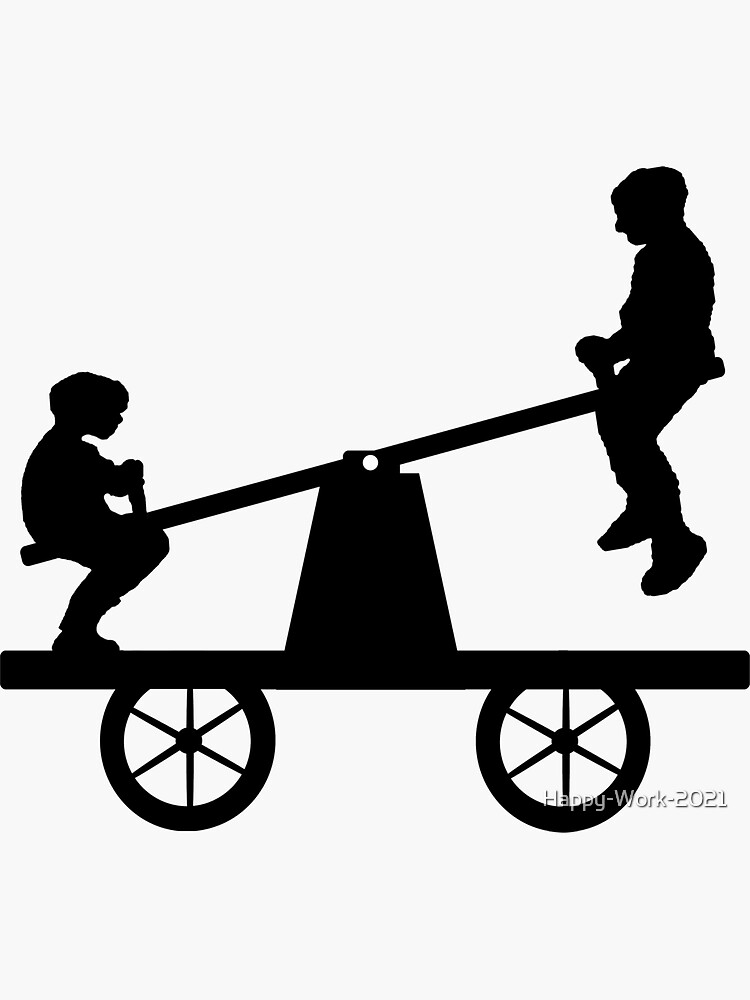The digital drawing is a detailed black-and-white line art illustration set against an off-white background. The image portrays a cart with two six-spoke wheels, resembling a rail cart, and features a seesaw mounted centrally on a triangular base atop the cart's flat platform. Two boys are depicted playing on the seesaw in profile and silhouette – the younger boy on the left is at the bottom position with his knees bent, while the older boy on the right is elevated with his legs dangling. The entire scene is rendered in black, creating a shadow effect against the light gray background. In the bottom right corner, white lettering reads "Happy-Work-2021." The illustration emphasizes both the whimsical movement of the seesaw and the nostalgic simplicity of the silhouette art style.